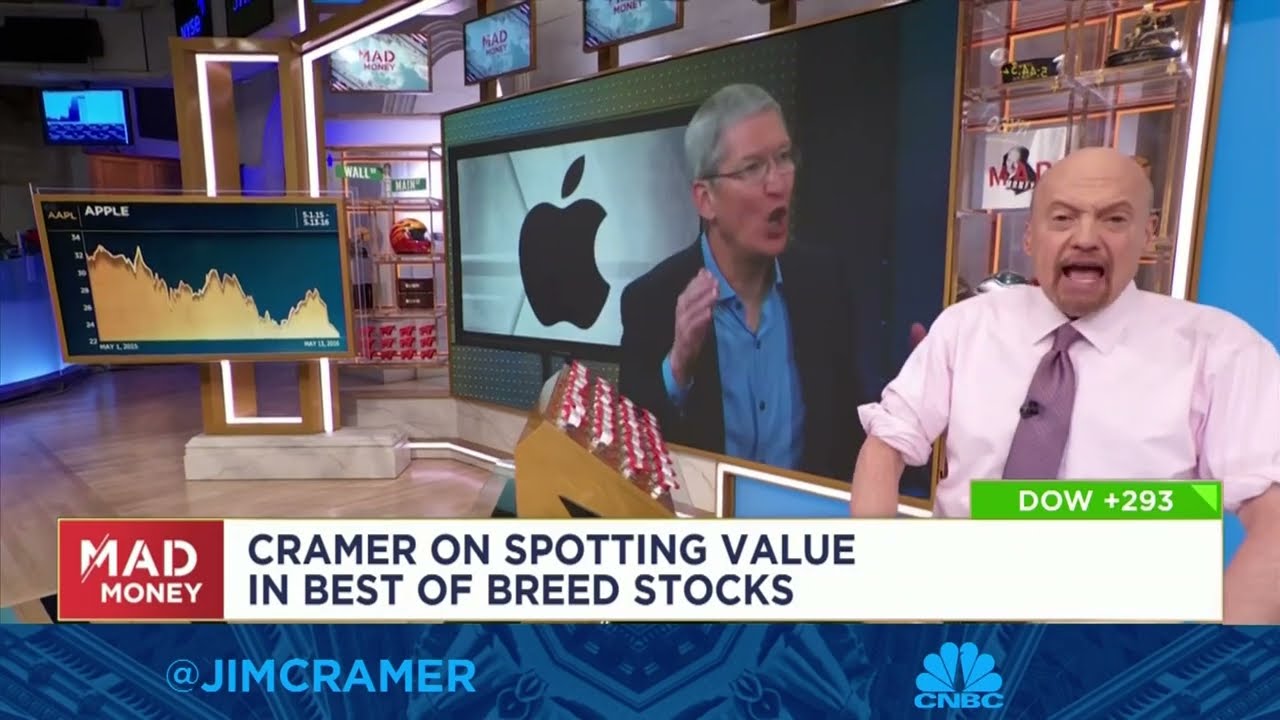The image is a detailed freeze-frame from a broadcast of CNBC's financial program "Mad Money" featuring Jim Cramer. The scene is set against a blue background and prominently displays the show's branding throughout. Jim Cramer, a bald man with a mustache, is positioned on the right side of the image. He is animatedly speaking to the camera, dressed in a pink dress shirt with the sleeves rolled up and a purplish tie.

At the bottom of the screen, a chyron in a red square box reads "Mad Money," followed by the text "Cramer on spotting value in best-of-breed stocks." Above this banner, a green box indicates "Dow Plus 293." Lower on the screen, a blue transparent band shows the hashtag @JimCramer alongside the CNBC peacock logo.

In the background, there are multiple screens associated with the show's set. One large screen prominently features Tim Cook, the CEO of Apple, giving a speech in front of the Apple logo. To the left is another screen displaying a chart illustrating Apple’s stock price history. Additional details include a window behind Cramer and a display case containing items such as street signs labeled "Wall" and "Main," and a helmet.